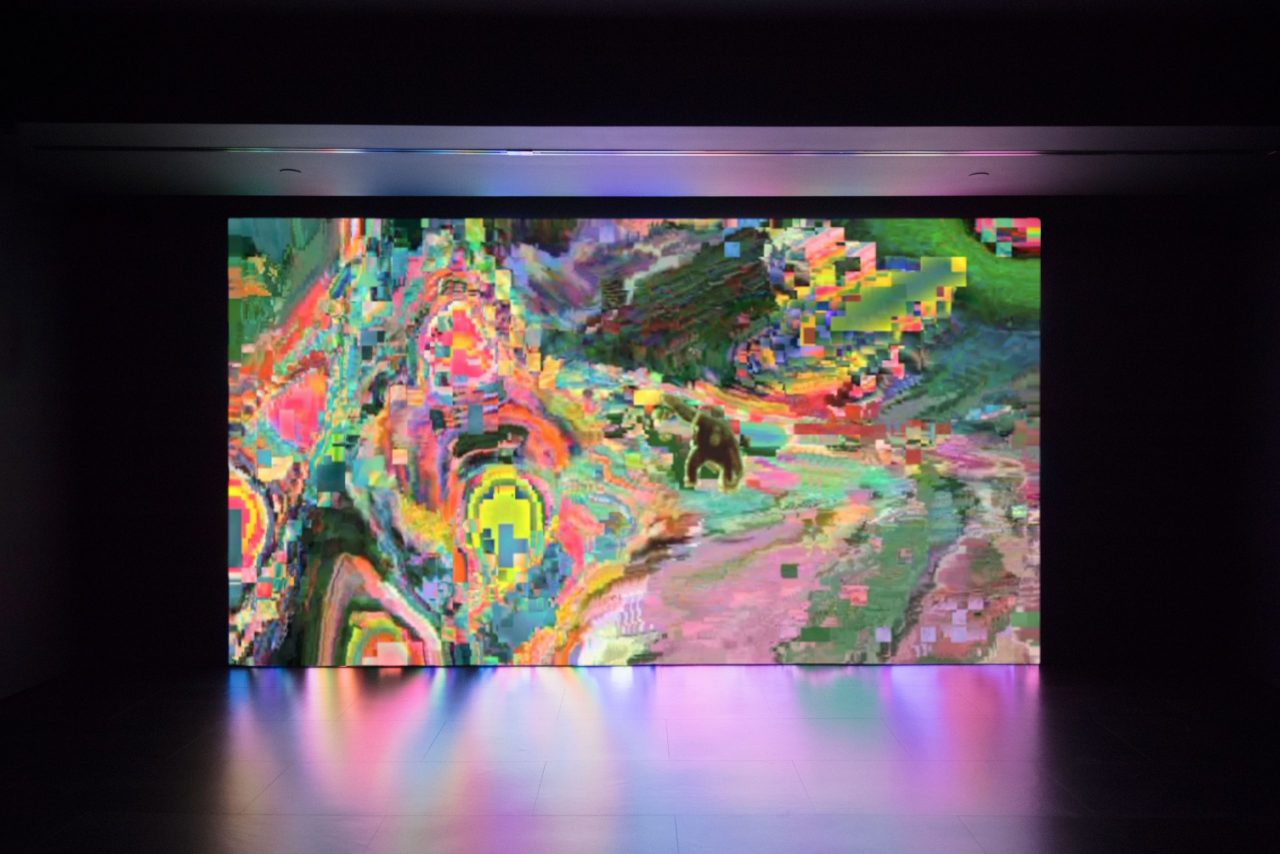In this image, there is a tall rectangular display screen centrally positioned in a very dark room, giving the setting a backlit appearance. The screen features an abstract, pixelated digital artwork which prominently displays a gorilla at its center. Surrounding the gorilla, the painting is vibrant and colorful, comprising swirling and blocky pixels in shades of yellow, pink, green, blue, red, and orange. At the top of the display screen, a metallic horizontal bar, silver in color with various reflections, can be seen, adding to the artistic ambiance. Below the screen, the surface reflects the colorful pixels, creating a crisp reflection that fades out gradually, contributing to an overall sense of depth. The background remains pitch black, with minimal visible details except for some recessed lighting or a rail on the ceiling, which catches the glow from the screen. The entire scene looks like a digitized painting, with a distinct, almost glitched texture that adds to its abstract and modern appeal.